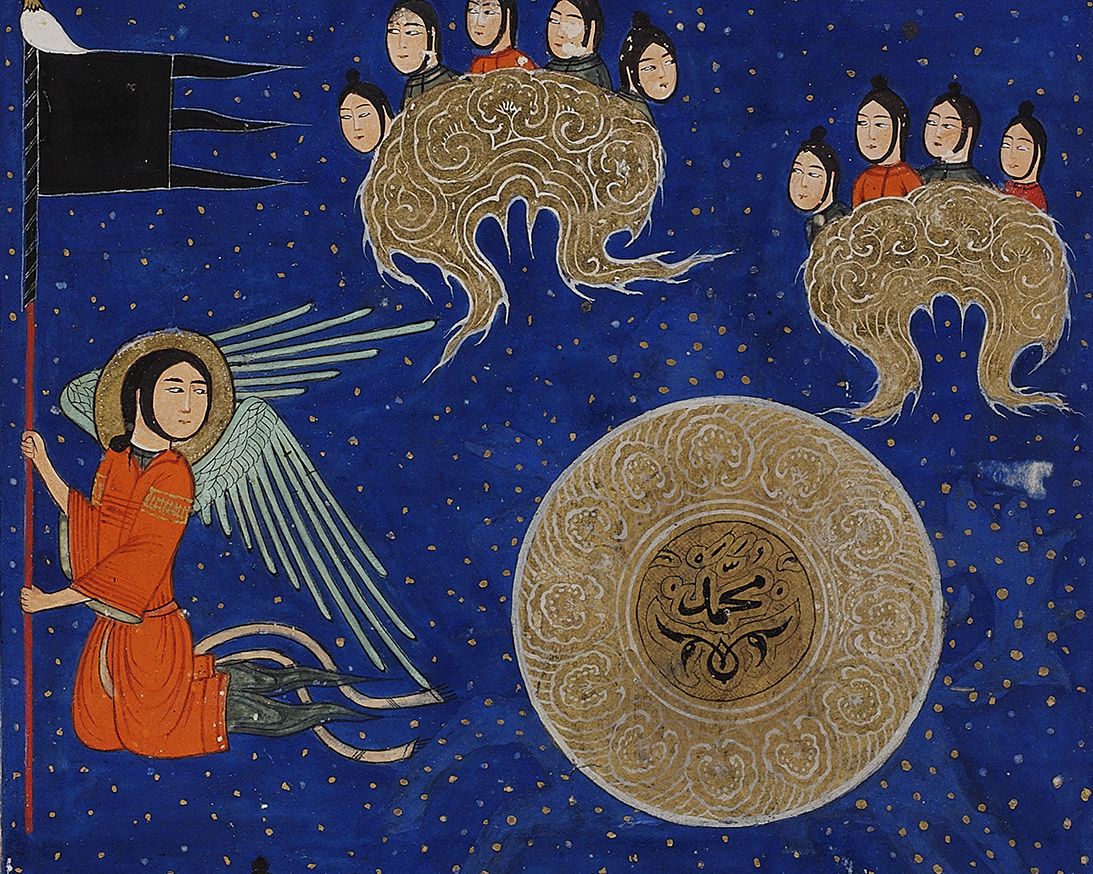The artwork is a detailed painting with Asian influences, prominently displaying a night blue sky dotted with numerous golden stars. Central to the image are multiple figures with dark hair, similar hairstyles, and a mix of red and black attire, either standing or seated on swirling, cloud-like objects of a brownish-yellow hue. In the bottom-left corner, there's an angelic figure dressed in an orange robe or kimono, distinguished by its wings and the absence of feet, trailing off into two flowing gray areas. This figure is holding a pole that ends with a black flag adorned with three trailing ribbons. Adjacent to the angel and occupying the upper middle section is a golden object with intricate swirl designs, supporting five individuals. Another similar object on the right holds four individuals. Towards the right side and lower in the composition, a prominent circular symbol is visible, featuring designs that resemble trees and additional patterns or letters within. The scene blends ethereal elements with traditional motifs, creating a harmonious yet mystical tableau.